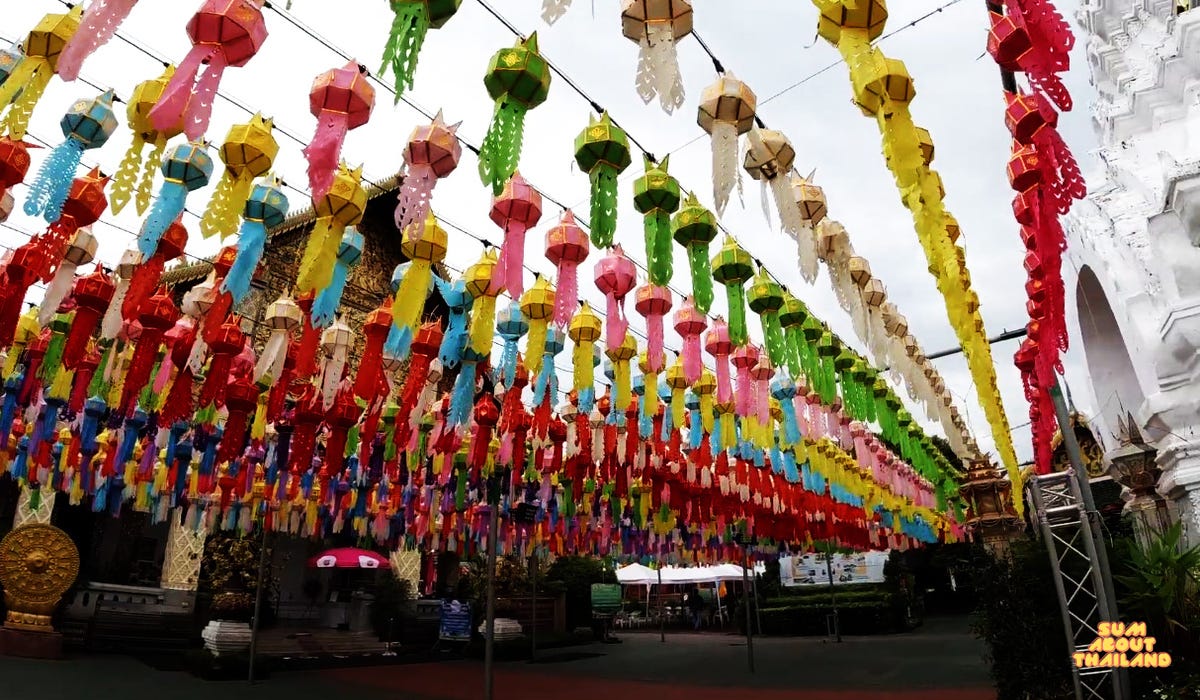The photograph vividly captures an outdoor market scene in Thailand, as hinted by the yellow text in the bottom right corner that reads "SUM about Thailand." The sky, clear yet overcast, provides a diffused light that illuminates the area without casting harsh shadows. Dominating the scene are hundreds of colorful lantern-like decorations strung across lines suspended in the sky. These decorations, resembling piñatas or intricate paper lanterns, are meticulously arranged in rows, each row showcasing a single color: red, yellow, white, green, pink, baby blue, and multicolored variations. The decorations extend deep into the background, creating a visually striking canopy of color. 

To the right, a large white stone building, akin to a temple, peeks into the frame, while the left features smaller beige structures that appear to house market stalls. A red umbrella, possibly for seating or shading merchandise, adds to the bustling ambiance. Although the ground color is difficult to discern, it complements the dark gray tones seen at the bottom of the image, likely indicative of pavement or concrete. Overall, the photo encapsulates the vibrant and meticulous preparations for what seems to be a large festival or celebration.